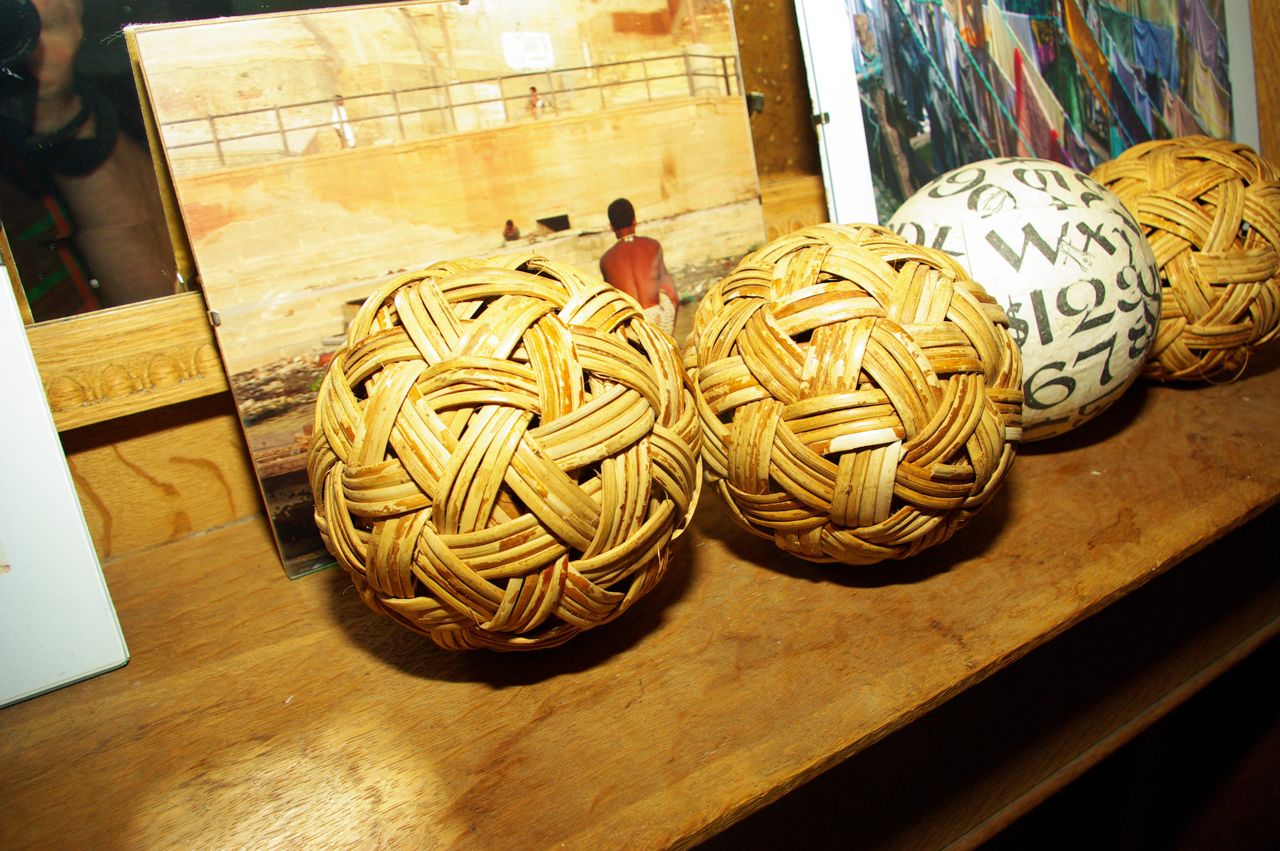A detailed photograph captures a light brown wooden table with natural patterns, resembling oak or pine. On top of the table sit four spherical objects: two woven wicker balls with intertwining straps, a third ball covered in white paper with black letters and numbers, and a fourth ball also displaying an intricate woven design. Positioned behind these objects are two pieces of artwork. On the left, a sepia-toned photograph shows a person standing facing a concrete wall with railings, while on the right, an abstract painting features vibrant blue, red, white, and orange streamlines enclosed in a white frame. The table's design includes a dark cubby space beneath its top surface without any visible contents.